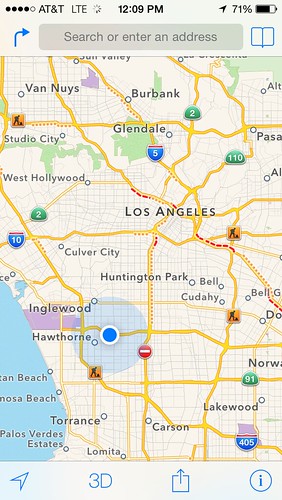The image is a screenshot from a cell phone displaying a map of the Los Angeles area. At the top-right corner of the screen, there is a battery symbol indicating 70% charge. Adjacent to this is the GPS location icon, an arrow slightly pointing to the upper right. Centered at the top is the time, which reads 12:09 PM. Moving to the left, there is the LTE symbol accompanied by a circular progress bar in motion, followed by the network provider, AT&T, and to the far left, the cell phone reception icon showing four out of five horizontal dots filled in. Below the status bar lies a search bar. The main section of the image is occupied by a detailed map showcasing various venues and cities within the Los Angeles area, including Burbank, Glendale, West Hollywood, Culver City, Huntington Park, Lakewood, Carson, Torrance, Inglewood, and Hawthorne.